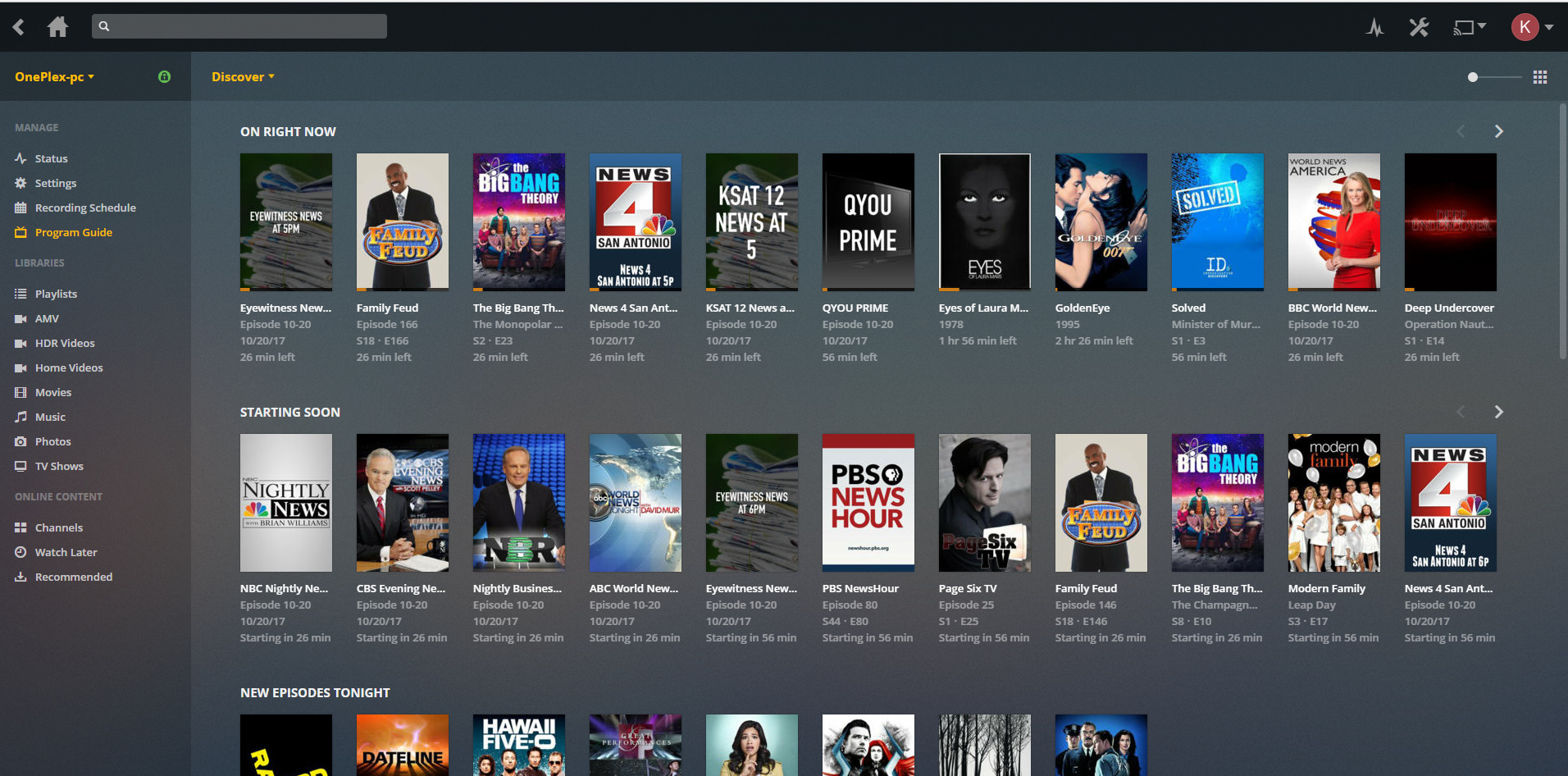The web page features a detailed layout with a blend of straightforward visual elements and essential information. A Caucasian individual is prominently positioned at the center, making direct eye contact with the viewer, creating a welcoming and engaging atmosphere.

The top left corner of the page is dedicated to contact details, including addresses, websites, and phone numbers, providing easy access to further information. The background consists of a predominantly singular color with subtle variations, and a computer or laptop component is faintly visible, suggesting a tech-oriented theme.

On the right side, a column lists various social media platforms such as Facebook, YouTube, and Twitter, indicating the page's connectivity and outreach capabilities. The bottom section features additional information about the services offered, ensuring that visitors have all the necessary details at their fingertips. Overall, the webpage is user-friendly with a well-organized structure that prioritizes accessibility and clarity.